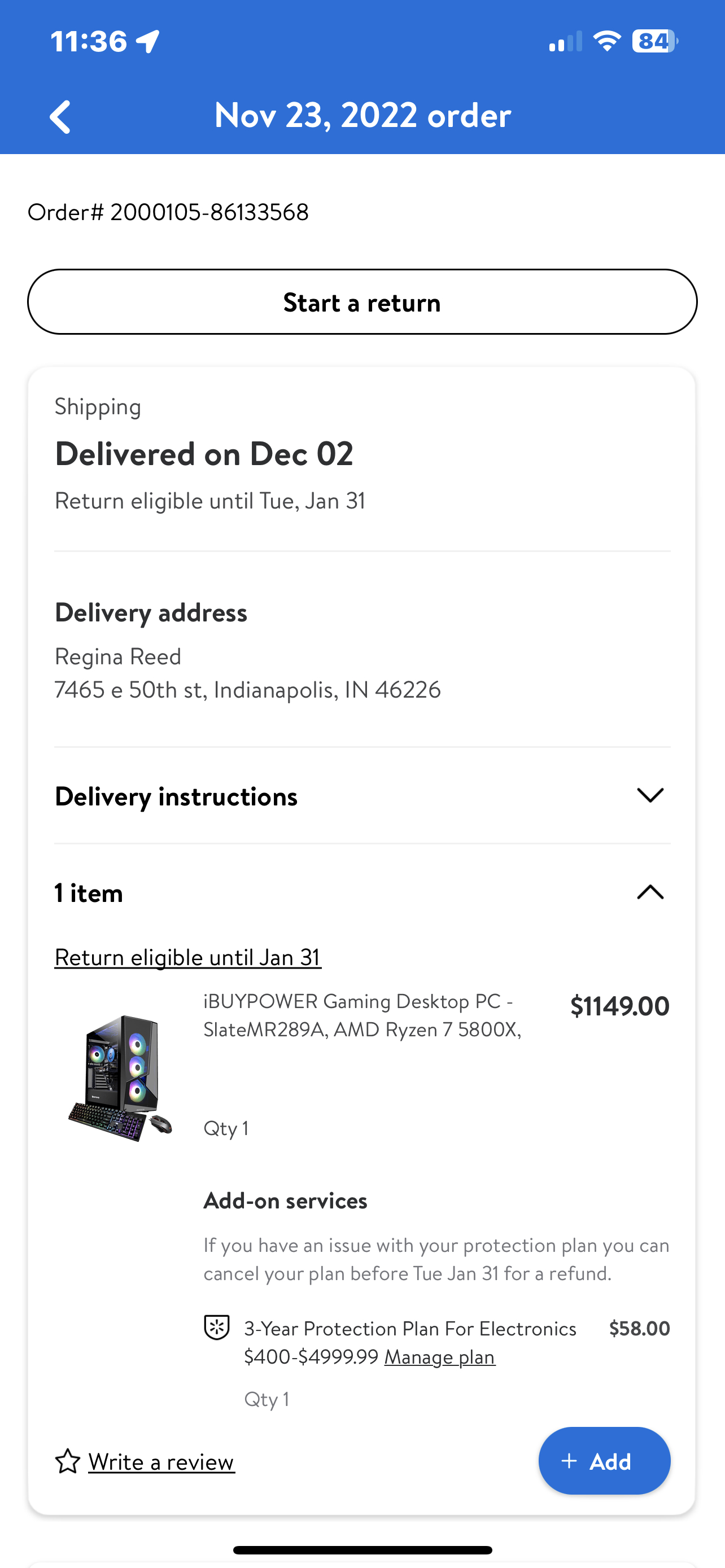This image is a detailed screenshot from a cell phone displaying an order summary. The top of the screen features a blue banner with white text, indicating that the time is 11:36 and the device is connected to Wi-Fi. The battery is at 84%, and there are two signal bars visible. The date is November 23rd, 2022.

The order summary includes:
- **Order Number:** Listed prominently, though the specific number is not provided.
- **Return Options:** A button to initiate a return.
- **Shipping Details:** It categorizes shipping information and notes that the package was delivered on December 2nd. The return is eligible until Tuesday, January 31st.
- **Delivery Address:** Regina Reed, 4765 East 50th Street, Indianapolis, Indiana 46226.
- **Drop-down Menu:** Provides additional delivery instructions.
- **Order Item:** Specifies one item, an iBUYPOWER gaming desktop PC.
- **Price:** $1,149.
- **Add-on Services:** Options for supplementary services.

The background of the image is white, with black text. The options and titles are highlighted in blue. An additional blue option includes an "Add" button accompanied by a plus symbol.

This comprehensive screenshot captures the order history of Regina Reed, specifically documenting her purchase of a gaming desktop PC.